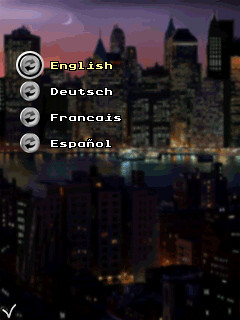The image depicts a vibrant cityscape at twilight, featuring a striking sky adorned with pink and purple hues and a crescent moon situated in the upper left-hand corner. The city is composed of numerous skyscrapers and smaller buildings separated by a shimmering body of water, highlighted by the numerous lights lining the water's edge. A couple of boats float peacefully on the water. On the left side of the image, there's a language selection menu comprising four buttons labeled English, Deutsch, Français, and Español. Each button features arrows pointing left and right, resembling a circular navigation. The currently selected language is highlighted with a yellow border, while the others remain white. Additionally, a checkmark is visible in the lower left-hand corner, suggesting a possibly interactive element. The overall appearance might indicate that this image is part of a website interface or an entry page, offering users the option to choose their preferred language.